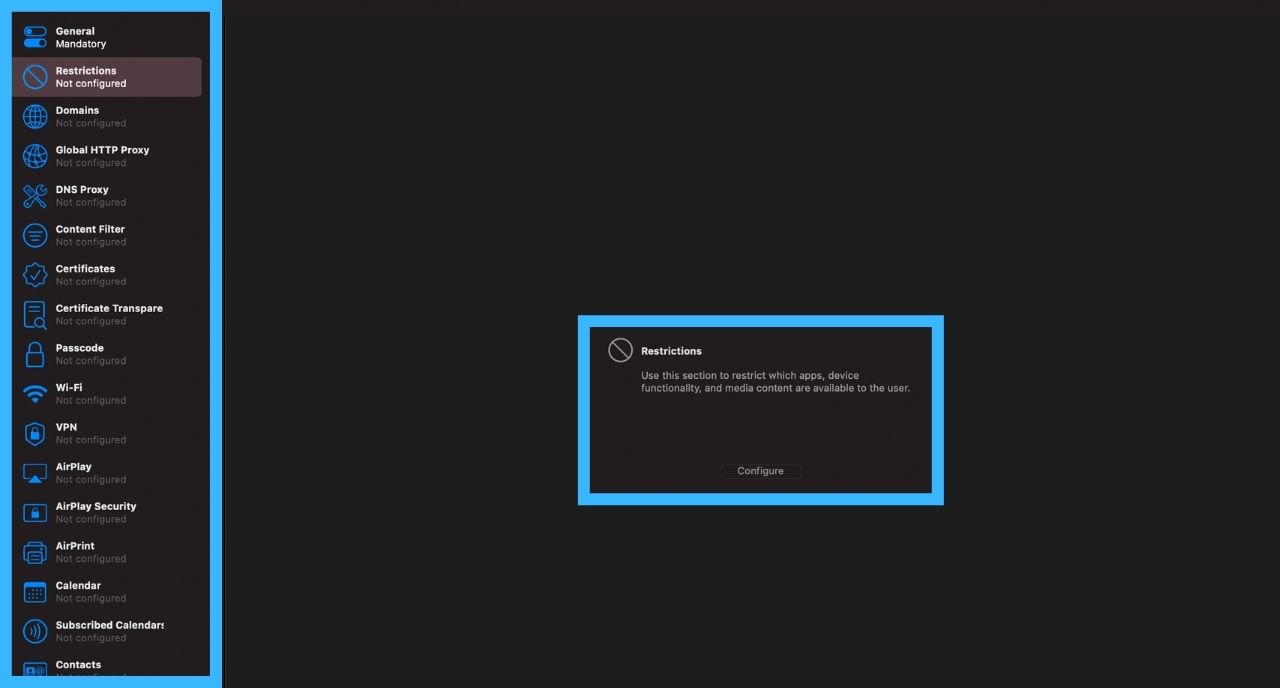The image captures a computer screen displaying a webpage with a predominantly dark black background. At the center of the screen lies a prominent, light royal blue rectangle, which is accompanied by a white circle with a slash icon and the word "Restrictions" in white text. Below this, a gray text box provides further details, stating, "Use this section to restrict which apps, device functionality, and media content are available to the user." 

A substantial space separates this information from a "Configure" button located at the bottom of the screen.

On the left side of the screen is a vertical toolbar featuring icons, each with accompanying text. The topmost icon, which is highlighted, represents "Restrictions" and indicates that restrictions are "Not configured." The following items on the list include a globe icon labeled "Domains," another globe icon labeled "Global HTTP Proxy," a set of tools labeled "DNS Proxy," an icon with a circle and lines labeled "Content Filter," a circle with a checkmark labeled "Certificates," and finally, a paper icon with a magnifying glass labeled "Certificate Transpire." The list continues in the same detailed manner down the page.